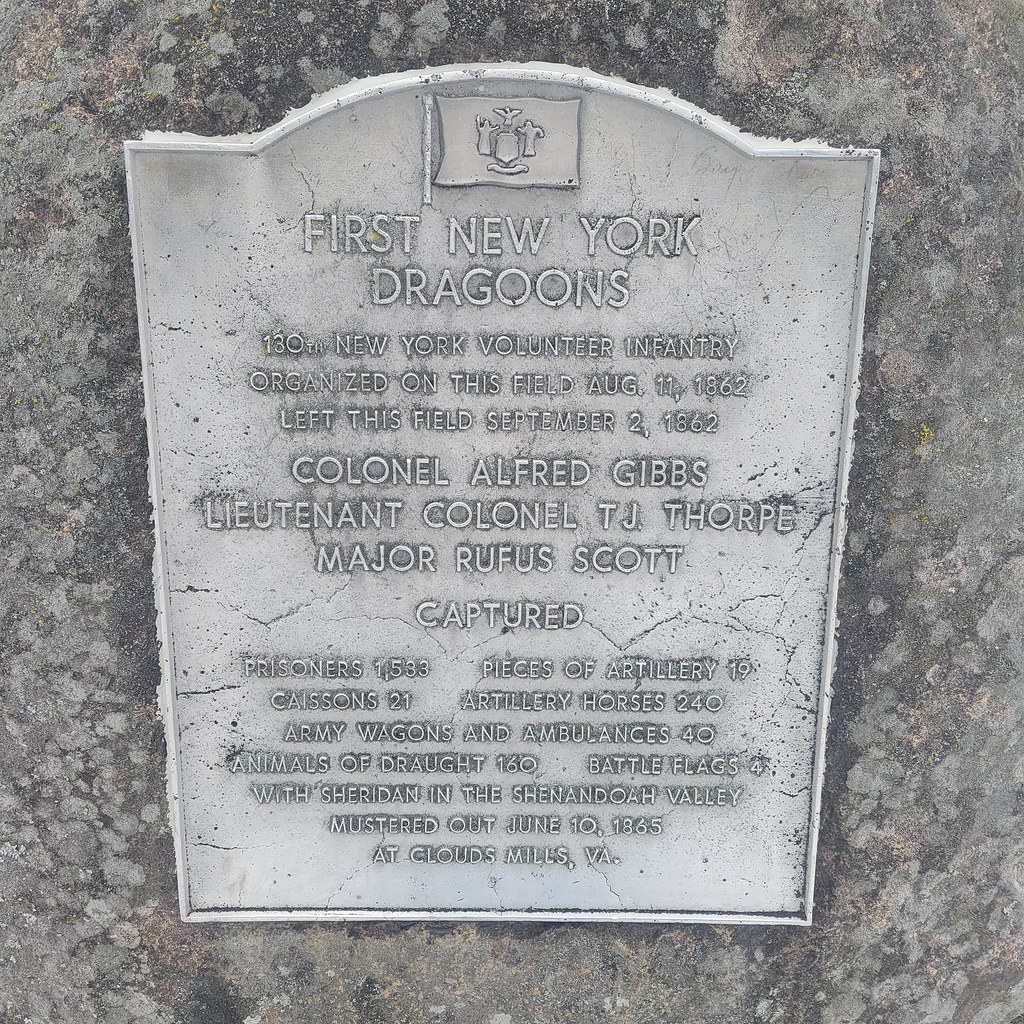This image features a detailed concrete monument with a silver plaque inscribed with historical information. At the top of the plaque, there is an insignia and a flag engraved, followed by the text "1st New York Dragoons" and "130th New York Volunteer Infantry." The inscription details that the infantry was organized on this field on August 11th, 1862, and left it on September 2nd, 1862. The names Colonel Alfred Gibbs, Lieutenant Colonel T.J. Thorpe, and Major Rufus Scott are listed alongside the word "captured." The plaque further enumerates the regiment's achievements: capturing 1,533 prisoners, 19 pieces of artillery, 21 caissons, 240 artillery horses, 40 army wagons and ambulances, and 160 draft animals, as well as capturing 4 battle flags. It also notes their involvement with Sheridan in the Shenandoah Valley. The regiment was mustered out on June 10th, 1865, at Clouds Mills, Virginia.